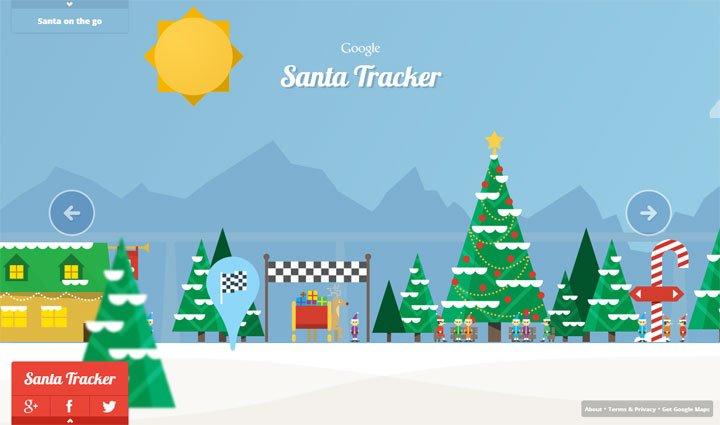This detailed and descriptive caption explains and contextualizes the visual elements present in the image to help the reader understand not just the content but also the setting and interactive components of the web page.

---

This image, sourced from a webpage featuring a Santa tracker, showcases a festive scene prominently branded with Google's logo at the top. The words "Santa Tracker" are displayed, emphasizing the holiday theme. The background is a picturesque winter landscape filled with numerous snow-dusted Christmas trees adorned with red ornaments. Towards the middle-right section of the image, a star-topped tree stands out prominently.

In the background, partially obscured by misty, overcast skies, mountains rise up, adding a sense of depth and seasonal chill to the scene. A radiant sun can be seen breaking through the clouds, enhancing the winter wonderland ambiance. Navigation buttons – a left-pointing arrow on the left and a right-pointing arrow on the right – suggest that the viewer can scroll through additional images or scenes.

Scattered throughout the scene are people dressed as cheerful elves, adding a playful element to the image. A reindeer, ready for holiday deliveries, stands next to a sleigh brimming with packages. A cozy house nestled among the trees and mountains further amplifies the festive spirit. At the top of the image, the phrase "Santa on the go" suggests an active, ongoing tracking experience. In the lower right-hand corner, options such as "About," "Terms and Privacy," and "Get Google Maps" are available, indicating additional information and tools accessible to the viewer.